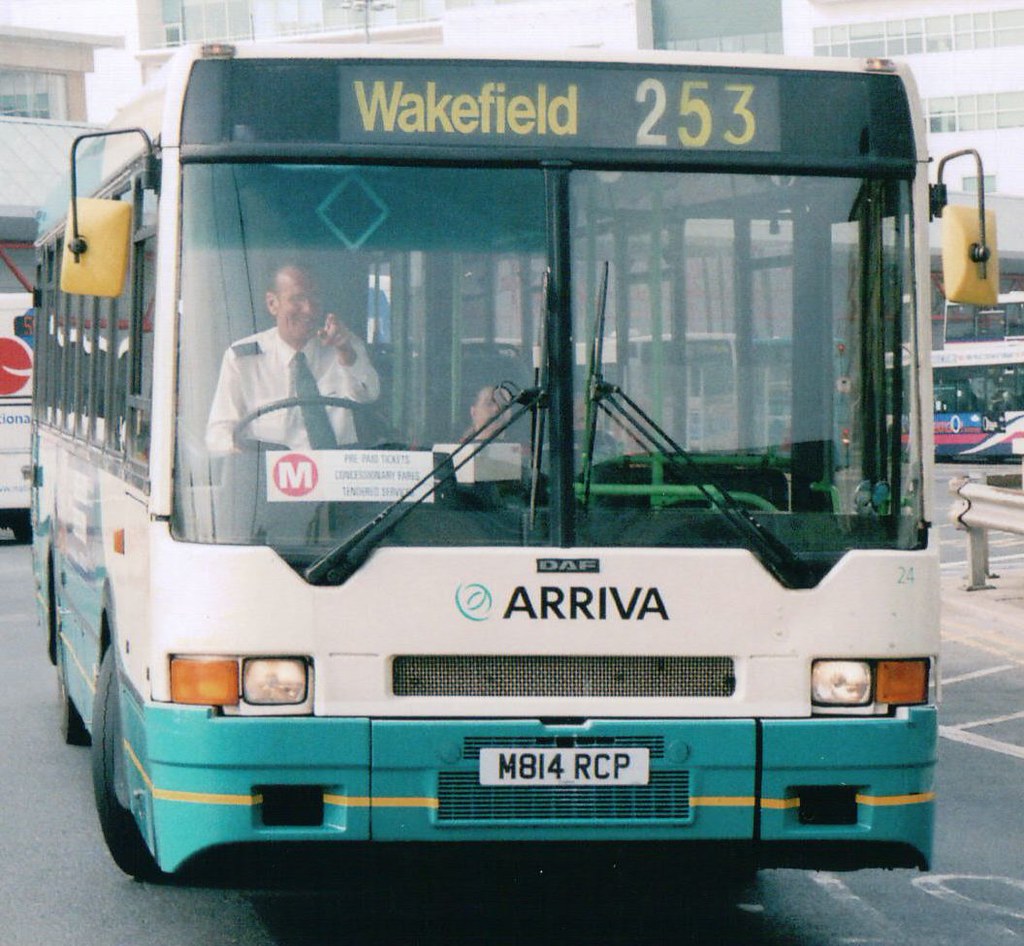The image depicts a city transit bus, likely located in England, given that the driver is seated on the right side. The bus has a flat front with a sign above the windshield displaying "Wakefield 253," indicating the route number. Below the windshield, in the center, is the word "Arriva," associated with the DAF emblem, suggesting the manufacturer. The bus features a European license plate reading "M814 RCP."

The driver, a white male wearing a white button-down uniform with a tie, is on the left side and appears to be smiling and pointing directly at the camera. The bus's exterior design includes a contrasting color scheme: the top half is white, while the lower half around the tires and bumper is a teal green, accented by a yellow stripe. Surrounding the bus, the scene captures an urban environment with other buses, cars, and buildings visible in the background.